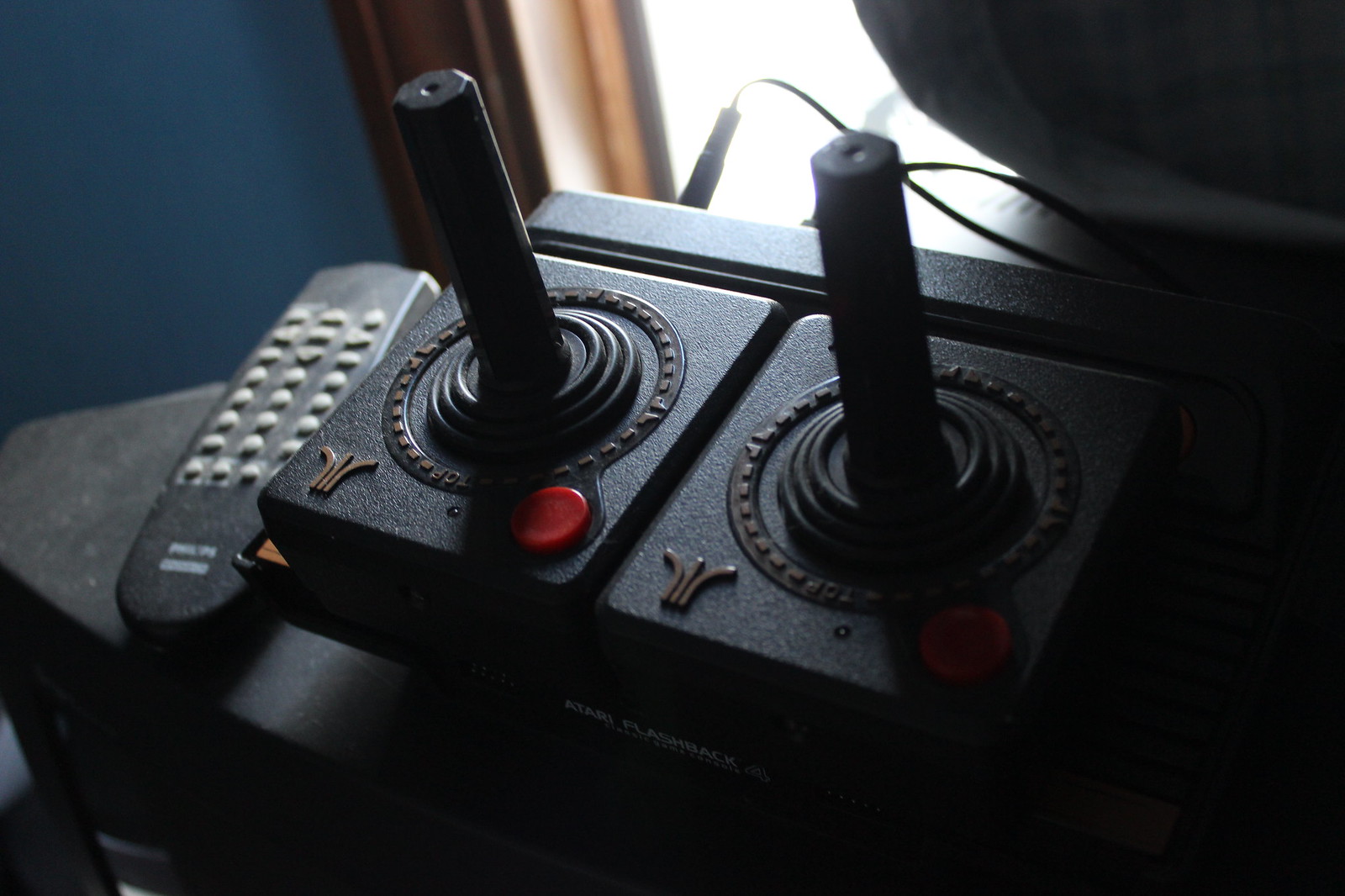This photograph captures a nostalgic setup featuring vintage Atari controllers and a Phillips TV remote control. The scene is somewhat dark, centered around two classic Atari joysticks placed side by side on what appears to be a black console or table. The joysticks are black, with straight joystick posts that fit into a concentric circle made of rubberized material. Each joystick features an Atari logo in the upper left corner and a prominent red button. The controllers are labeled with "Atari Flashback" and seem to be inserted into an Atari console system.

To the left of the joysticks, a TV remote control branded "Philips" is visible. The background reveals a navy blue wall with stained brown wooden trim outlining a window. The window streams in blown-out white light, adding a stark contrast to the dimly lit room. Also partially visible to the right of the window is a piece of buffalo-checked gray curtain, completing the rustic ambiance of the scene.